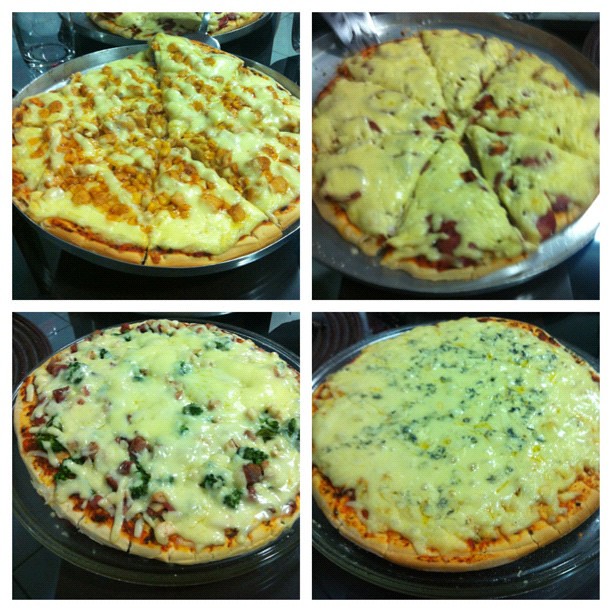This image is a composite photograph divided into four quadrants by a white cross, each quadrant depicting a different pizza. The pizzas are placed on either round metal or black pans. In the upper left quadrant, there's a thick and fluffy pizza loaded with melted cheese and topped with what appears to be bacon or hamburger. The upper right quadrant shows another pizza heavily laden with cheese, its exact toppings obscured but featuring a well-baked crust. The bottom left quadrant displays a cheese-covered pizza with visible green toppings, likely spinach or other green vegetables. Lastly, the bottom right quadrant includes a pizza with lots of white melted cheese and sprinkled green herbs. Each pizza features a substantial crust, with the overall image slightly blurry and unenhanced, emphasizing the abundance of cheese and varying toppings.